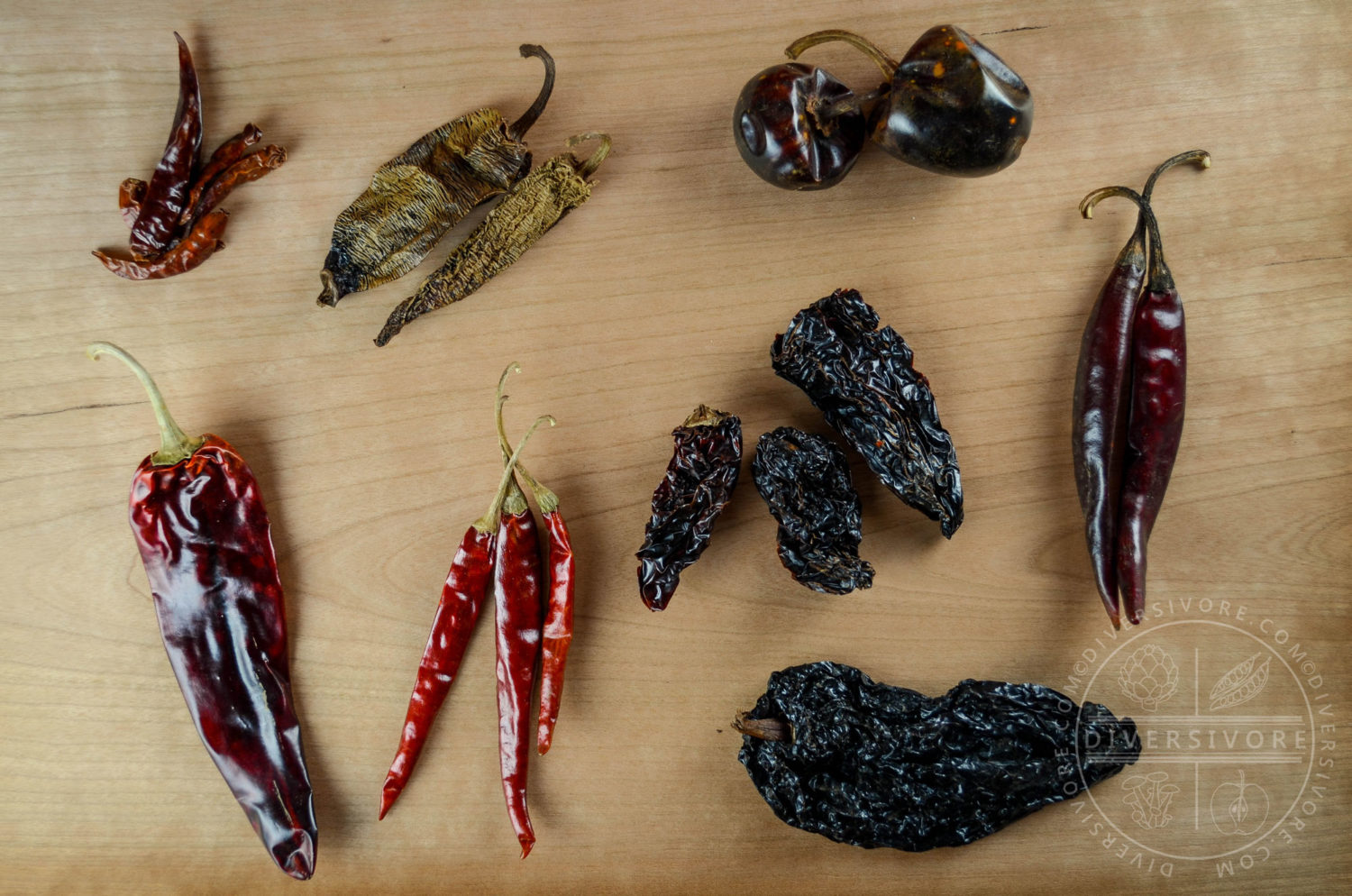The image displays an assortment of eight distinct varieties of dried peppers arranged on a brown-tan wooden table, showcasing the natural grains of the wood. Starting from the upper left, there is a tiny, skinny, reddish-orange chili with an elongated shape. Next to it is a dried pepper reminiscent of a jalapeno or serrano, displaying a light whitish-green skin. The third pepper is shaped like a small berry, exhibiting dark, nearly black coloration with brownish-red tones and a poofy appearance.

Moving to the bottom row, the first pepper is a large, shiny, burgundy-red variety with a long form and prominent stems. Beside it are three long, skinny, vibrant red chilies. Further along are four shriveled, black peppers with a texture resembling raisins, which are likely ancho chilies. Lastly, there are two long, dark cherry-red chilies, completing the vibrant and diverse display. In the lower right corner of the image, the logo for the company "Diversivore" is visible.